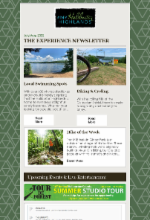This image appears to be a snapshot of a webpage, likely from a travel website or a digital brochure promoting various tourist destinations. The borders of the page are filled with forest green patterns interspersed with white designs, adding a naturalistic touch to the webpage. 

At the top center of the page, a blurred heading reads "Experiences Newsletter," suggesting the content is an informative piece about travel experiences. Below this title are three primary images arranged in a grid. 

The first image captures the serene view of a lake with a sandy beach, likely a popular spot for relaxation and water-related activities. Adjacent to this, the second image displays a camping area, possibly showcasing tents and campfire settings that would appeal to outdoor enthusiasts.

In the lower center of the page, there is a picture of a person walking down a hiking trail. The hiker is wearing a distinctive red shirt, black pants, and hiking shoes, emphasizing the sense of adventure and exploration.

Finally, the bottom of the page features a banner ad which invites viewers to "Tour the Forest," and promotes a "Summer's Studio Tour," highlighting a specific seasonal event or guided tour option.

Overall, the webpage is designed to captivate and inform potential travelers about various recreational areas and activities.